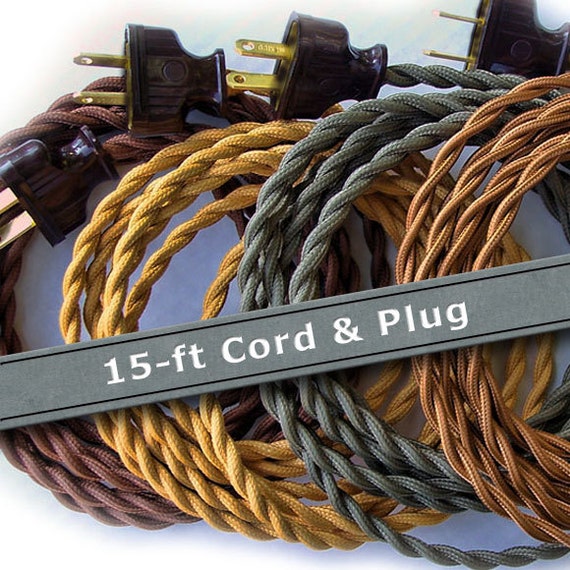The large square image vividly illustrates four coils of cords, each uniquely colored and materialized, overlapping in a mesmerizing arrangement. Dominantly centered across the image, a gray horizontal rectangle bears the white text "15-FT CORD AND PLUG," creating a stark contrast and clear emphasis. These cords, coiled in an almost circular shape, exhibit a spectrum of colors and textures: a medium brown cord on the left, followed by a gray cord towards the center, a lighter brown cord adjacent to it, and a burgundy braided cord at the bottom. Each cord culminates in a black-based plug with two protruding gold prongs, all uniformly facing left. Additionally, the cords appear to be constructed from various materials, suggesting differences in fabric or twine, with one described as potentially nylon. The intricate placement and diverse colors of the cords—ranging from yellow tan to rose gold hues—further enhance the intricate visual appeal, making each cord distinguishable and detailed.